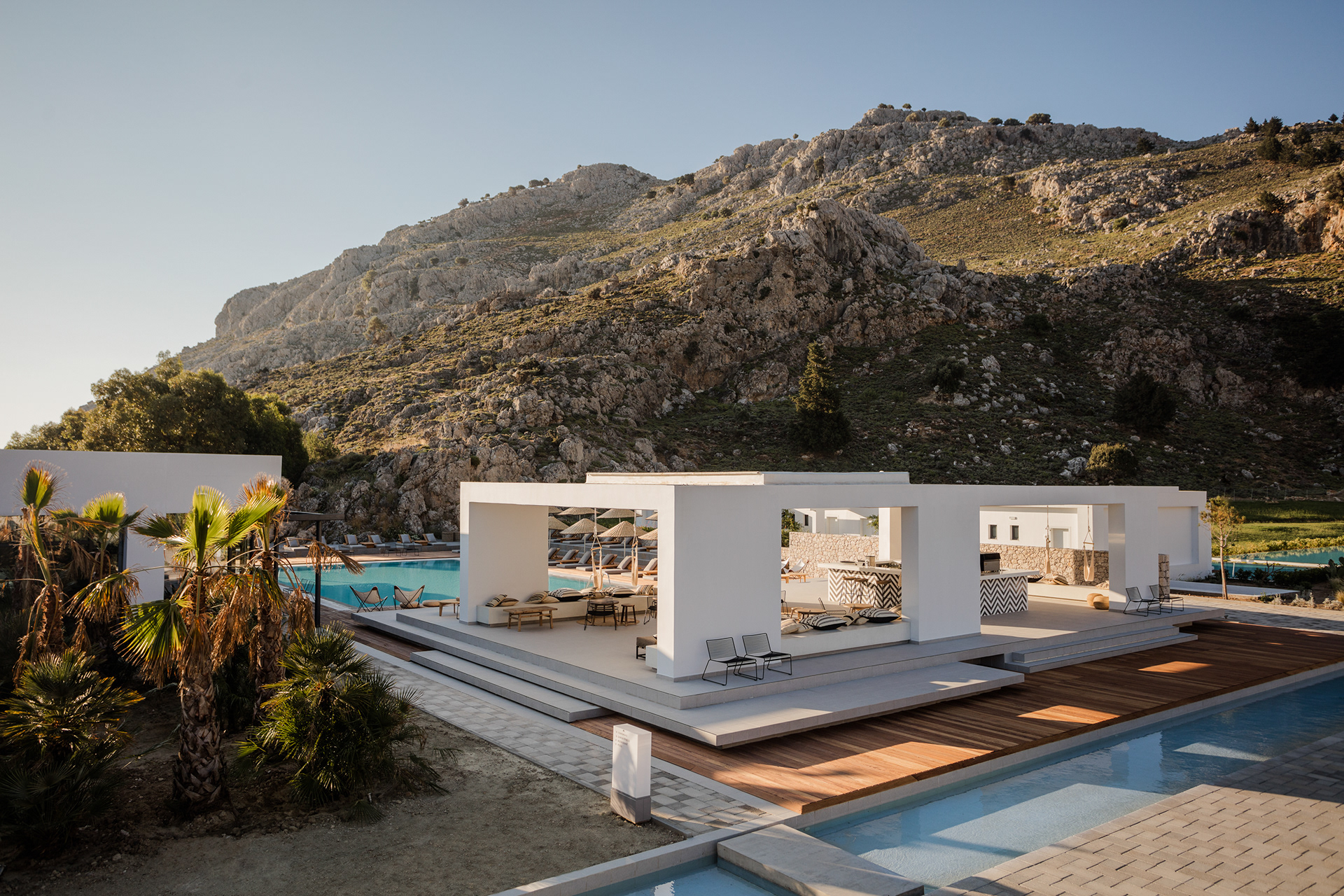The photograph showcases a high-end luxury villa nestled in an exotic, possibly tropical or arid location like Hawaii or a Greek island. The focal point is a pristine, white, stuccoed pavilion with a unique architectural design that is low, flat, and geometric. This open-air dwelling has partial walls but no windows, creating a seamless connection with the surrounding elements. The structure appears slightly elevated, giving it a floating impression. Outdoor furniture is arranged underneath the pavilion, providing a shaded area to relax. In the foreground, a rectangular or square-shaped swimming pool is present, while a channel of water runs along the front of the building, adding to the serene atmosphere. To the right and left, additional buildings partially obscured by lush palm trees can be seen. The backdrop features a rugged mountain range with a rough, lava-like texture, enhancing the natural beauty of the setting. This exquisite location exudes a resort-like ambiance, ideal for special occasions such as weddings or honeymoons.